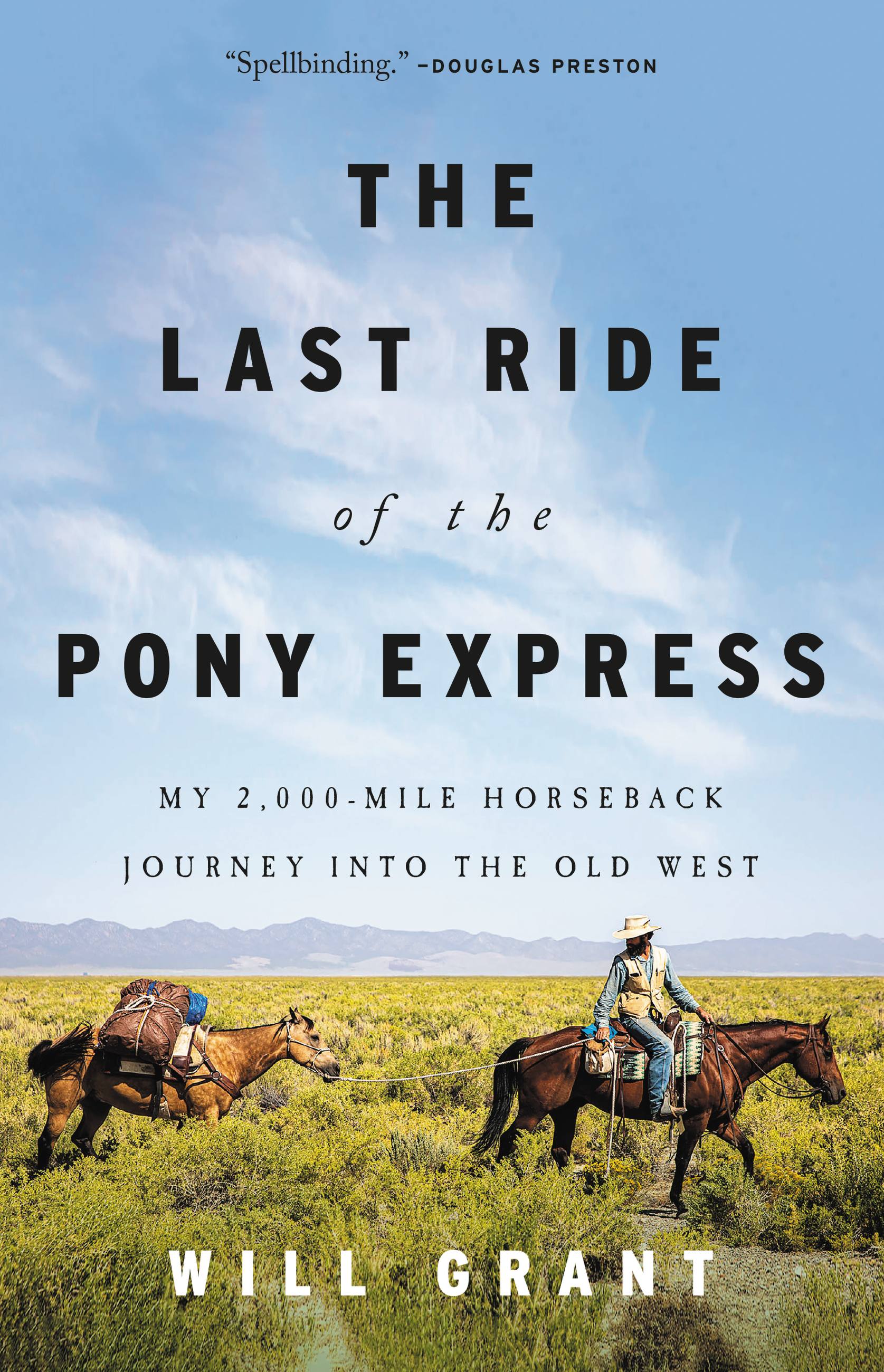The cover of the book "The Last Ride of the Pony Express: My 2,000 Mile Horseback Journey into the Old West" by Will Grant features a vivid and detailed illustration. The background showcases a blue sky with thin, scattered white clouds, extending down to a distant horizon marked by faint mountains. The foreground is a sprawling field of light yellowish-green grass and bushes.

Dominating the right side of the image is a cowboy, dressed in blue jeans, a tan vest, a blue shirt, and a cowboy hat. He is mounted on a brown horse, with one leg lifted as if in motion. In his right hand, he holds a rope or lasso, which is tethered to a second horse behind him. This pack horse is a lighter, golden-brown color and is laden with supplies, including a brown bag and a blue bag.

At the top of the cover, a quote from Douglas Preston reads, "Spellbinding," lending acclaim to the book. The title, "The Last Ride of the Pony Express," is prominently displayed in large black letters, with a subtitle in smaller type detailing the author's adventurous journey. At the bottom in white letters is the author's name, Will Grant. This evocative image perfectly encapsulates the rugged spirit and historical journey of the Pony Express.